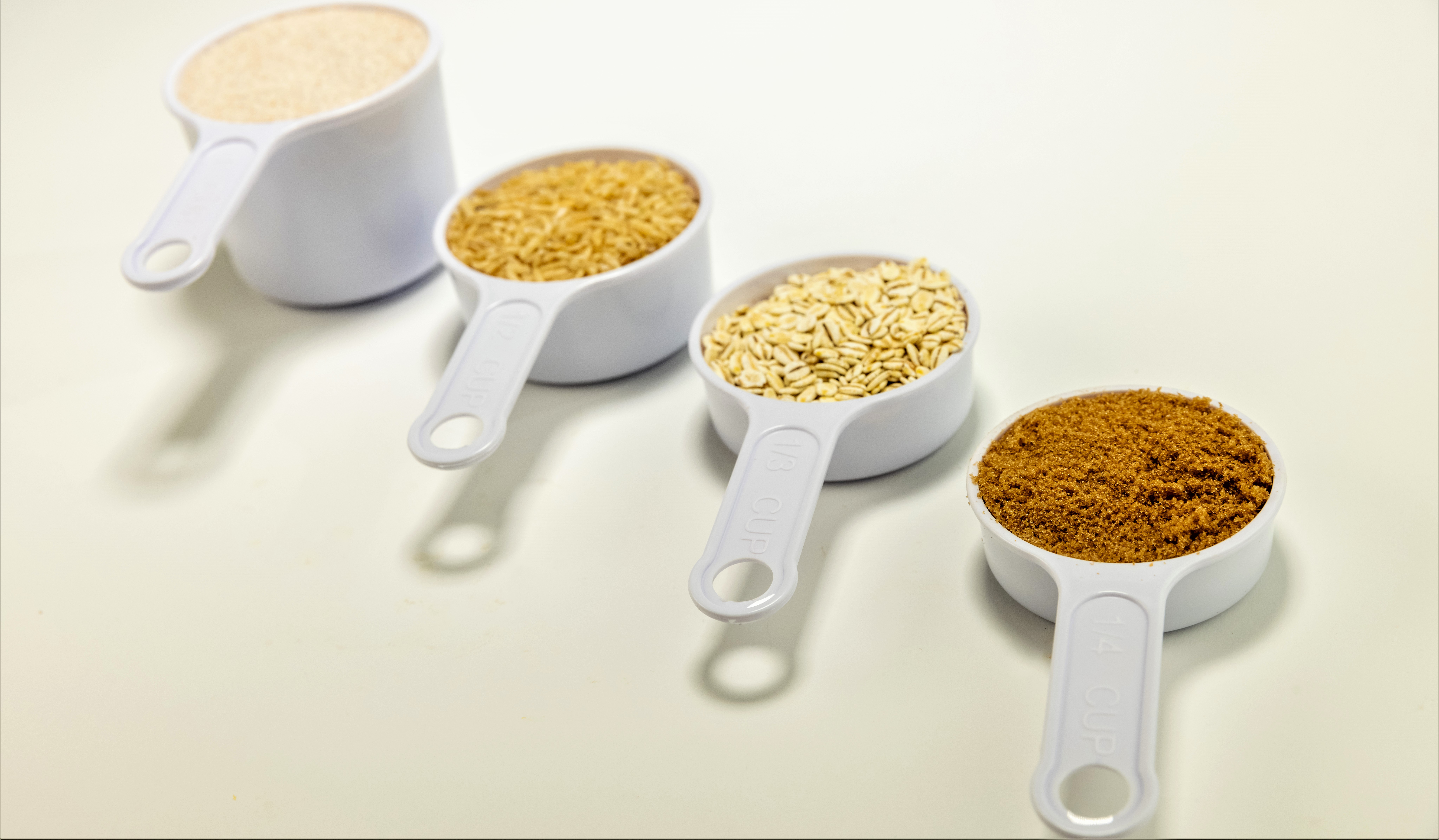The image is a color photograph taken in what appears to be a kitchen or pantry, featuring four white plastic measuring cups arranged in a lineup from largest to smallest. The largest cup, positioned at the top left, contains a creamy-colored substance, possibly dip or cream. The second cup from the left appears to hold yellow seeds, while the third cup, second from the right, contains white seeds. The smallest cup, situated at the bottom right, is filled with brown sugar. Each cup is clearly labeled with measurements: one cup, half a cup, a third of a cup, and a quarter cup, respectively. They are placed on a white surface, casting slight shadows beneath their handles, adding to the detailed realism of the scene.